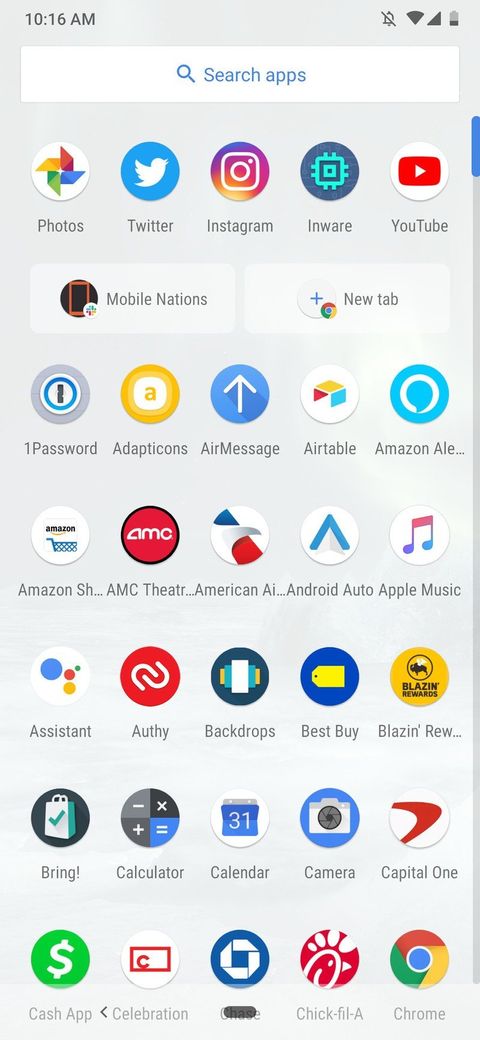This image displays a screenshot taken from a smartphone, which is set against a light gray background. In the upper left corner, the time reads "10:16 a.m." On the upper right side, various status icons are visible: notifications are turned off, Wi-Fi is enabled, full reception is indicated, and the battery icon shows a low charge. Beneath these icons is a white search bar with blue text, which reads "Search apps."

The main portion of the screenshot showcases a grid of app icons arranged in rows, each categorized from left to right as follows:

First row: 
- Google Photos
- Twitter
- Instagram
- inWare
- YouTube

Second row:
- Mobile Nations

Third row:
- 1Password
- Adapticons
- AirMessage
- Airtable
- Amazon Alexa

Fourth row:
- Amazon
- AMC Theaters
- American Airlines
- Android Auto
- Apple Music

Fifth row:
- Assistant
- Authy
- Backdrops
- Best Buy
- Blazin' Rewards

Sixth row:
- Bring!
- Calculator
- Calendar
- Camera
- Capital One

Each app icon is distinctly colored and shaped, lending a colorful and organized appearance to the phone's home screen. This detailed layout provides a comprehensive view of the user's frequently accessed applications.